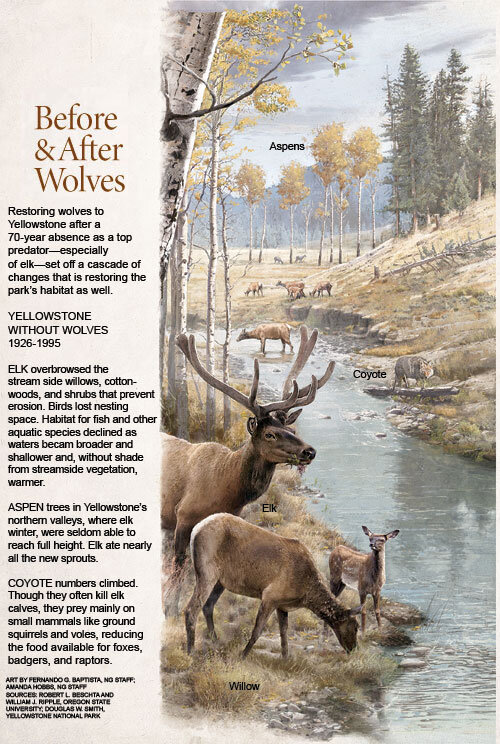The image resembles a rustic, vintage page from a book or wildlife magazine, primarily dedicated to the subject of wolves in Yellowstone. The layout is divided into two main sections: the left-hand side and the right-hand side. The left side features a light beige background with the prominent title "Before and After Wolves" in brown font, followed by several paragraphs of black text. This text provides detailed information about the reintroduction of wolves to Yellowstone after a 70-year absence, specifically highlighting the years 1926 to 1995, and discusses their impact on the ecosystem, mentioning elks, Aspen trees, and coyotes. It also includes credits for the artwork by Fernando Baptista and information on its originating university.

The right-hand side presents a scenic, muted illustration depicting a section of Yellowstone. The scene shows a variety of wildlife, including elk and deer, congregating by a flowing stream or river. In the background, there are green pine trees and some aspens with lighter, even white bark, and yellow leaves. Some of the trees have fallen, adding to the natural, untamed feel of the landscape. Labels in the image identify specific elements such as Aspens, Coyote, Elk, and Willow. Additionally, some distant animals are indistinct, contributing to the depth of the scene. The overall image exudes an old, slightly faded charm, capturing the serene, yet vibrant life amidst Yellowstone's varied habitat.